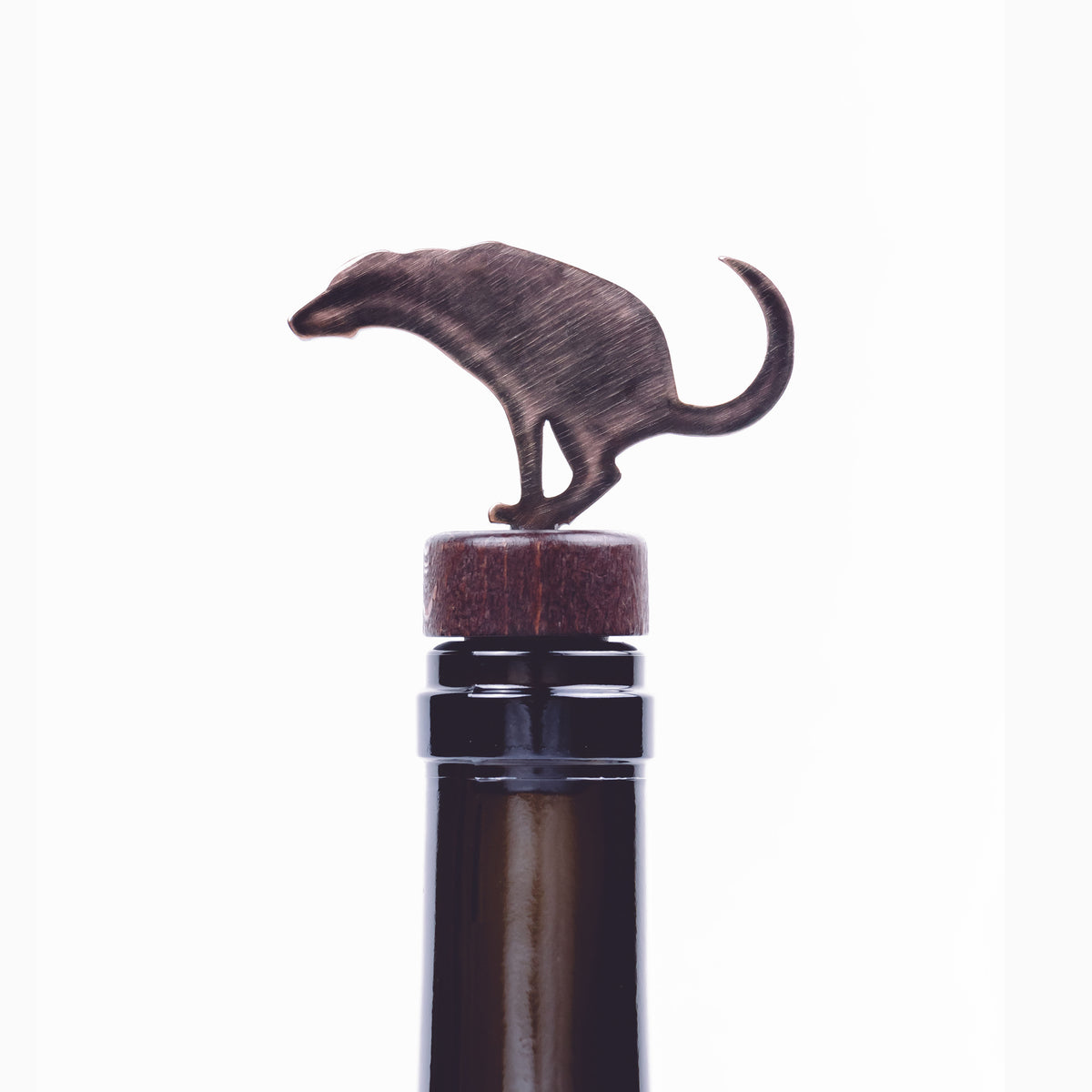This image features a humorous and uniquely designed wine bottle topper. The bottle itself is made of dark, possibly black glass, while the topper comprises a dark wooden cork adorned with a metal silhouette of a dog in a crouching position, resembling a dog trying to poop. The dog’s tail curves upwards like a crescent moon, and while it lacks detailed features, it captures the essence of a playful, hand-sculpted design. The snapshot is taken against a stark white background, devoid of any additional elements, bringing full focus to the whimsical bottle topper.